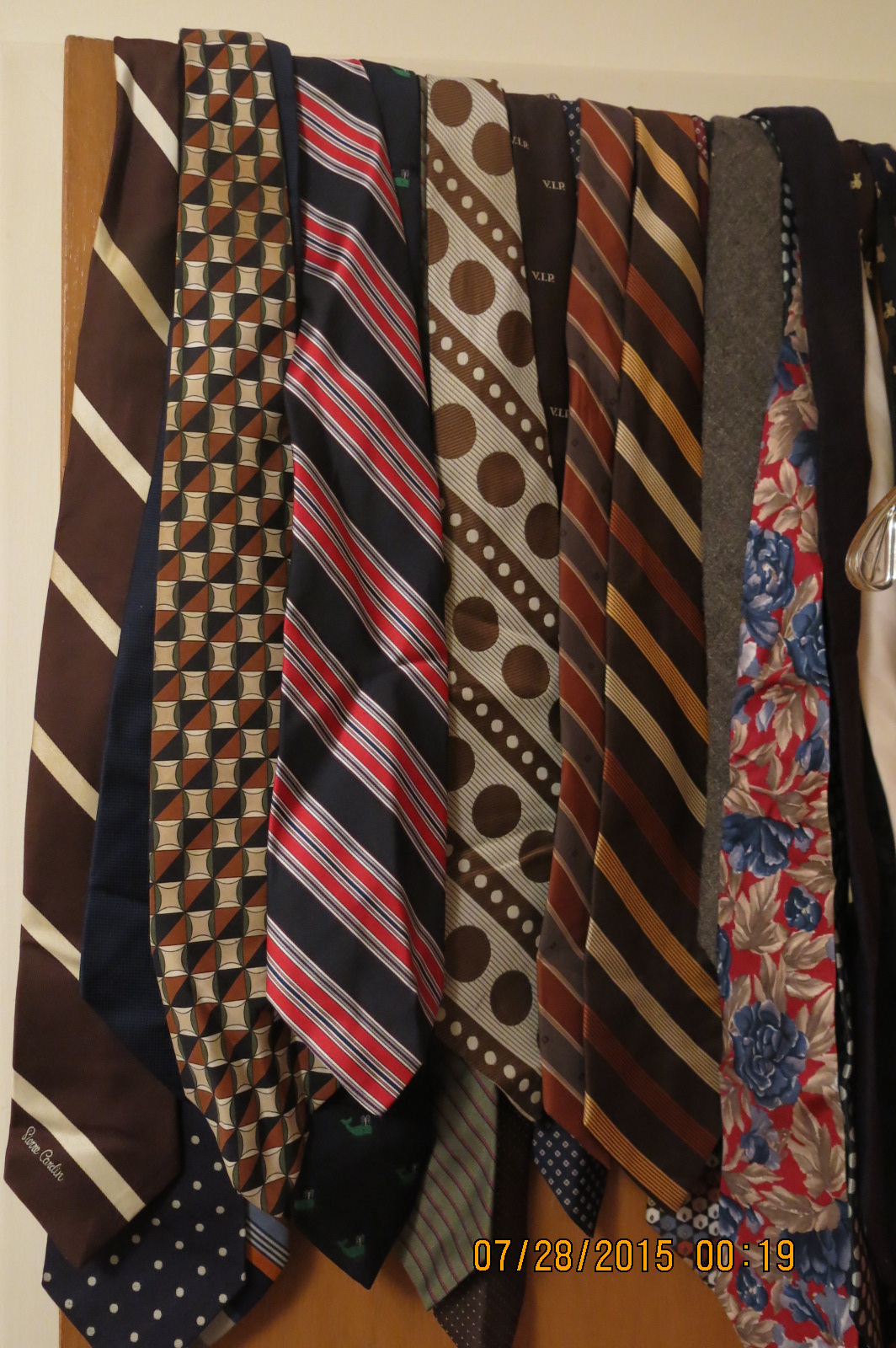The photograph features a collection of approximately 12 to 15 ties draped over the top of a medium brown wooden door set against a white wall. These ties exhibit a variety of colors and patterns, primarily within brown, blue, and cream color schemes. Notably, there is a brown tie with taupe diagonal stripes and a navy blue tie with white polka dots. A busy patterned tie with brown and black diagonally crossed squares interspersed with hourglass shapes stands out, along with a navy blue tie with diagonal red, black, and silver stripes. A blue tie with green dots, possibly depicting small figurines, further adds to the variety, accompanied by another blue polka-dotted tie. Additional ties include one with a white, taupe-ish background featuring polka dots and diagonal stripes, a brown tie labeled with "VIP", a red tie with blue flowers and silver-brown leaves, and several metallic-toned ties with maroon, gold, and bronze stripes. The texture of some ties appears felt-like and others silky. The date and timestamp on the bottom right corner indicate the photo was taken on July 28, 2015, at 12:19 AM, and a plastic hanger is visible among the ties on the right side.